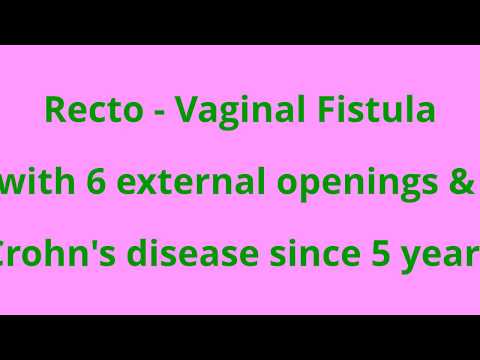The image appears to be a partial slide from a PowerPoint presentation, featuring text within a black frame on the top and bottom, reminiscent of a widescreen format. The background between the black bars is a pink rectangle. At the center of the image, in bold, green bubble lettering, the text reads: "Rectovaginal fistula with six external openings and Crohn's disease since five years." The text is cut off at the sides, implying that this is just a fragment of the full slide. The slide seems to detail a medical diagnosis, potentially as a post-exam summary, highlighting the condition and duration experienced by a person. The incomplete sentences and the cut-off edges suggest that the entire content is not fully visible in the image.